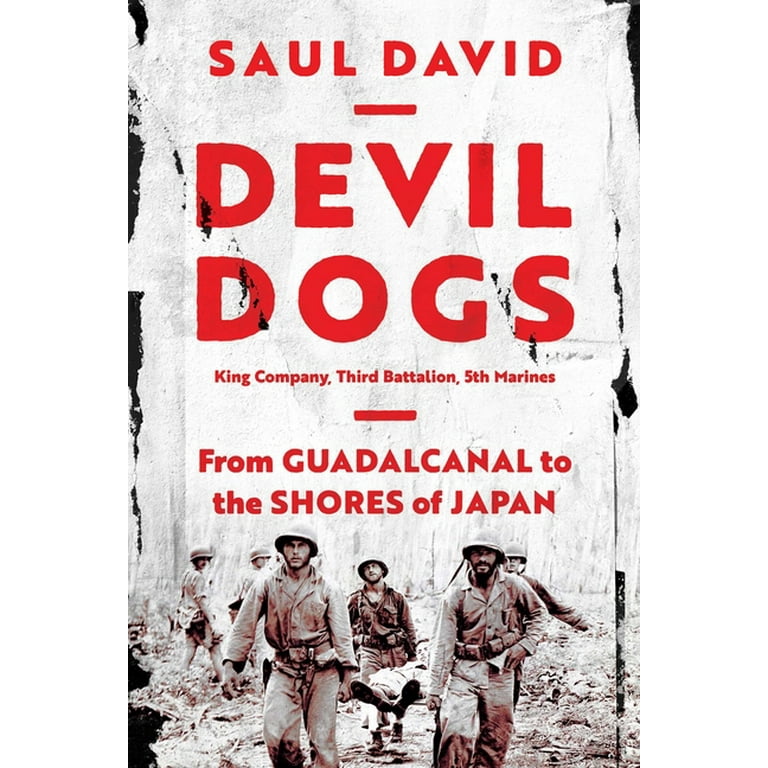The cover of the book, authored by Saul David and titled "Devil Dogs: King Company, 3rd Battalion, 5th Marines, From Guadalcanal to the Shores of Japan," features a rugged, worn white background overlaid with large, bold red text. The author's name, Saul David, appears at the top, followed by the title "Devil Dogs," with the subtitle positioned below in smaller text. The lower portion of the cover displays a sepia-toned photograph of seven soldiers in helmets and uniforms. Four of these soldiers are central in the image, carrying a gurney with an injured comrade, whose feet are visible towards the front. The two men positioned at the back and the two others on the left appear to be aiding or observing the situation. The backdrop suggests a jungle or battlefield, with various debris scattered on the ground, embodying the harrowing conditions faced by the Marines. The textured, distressed design of the cover reflects the gritty and intense nature of the book’s content.